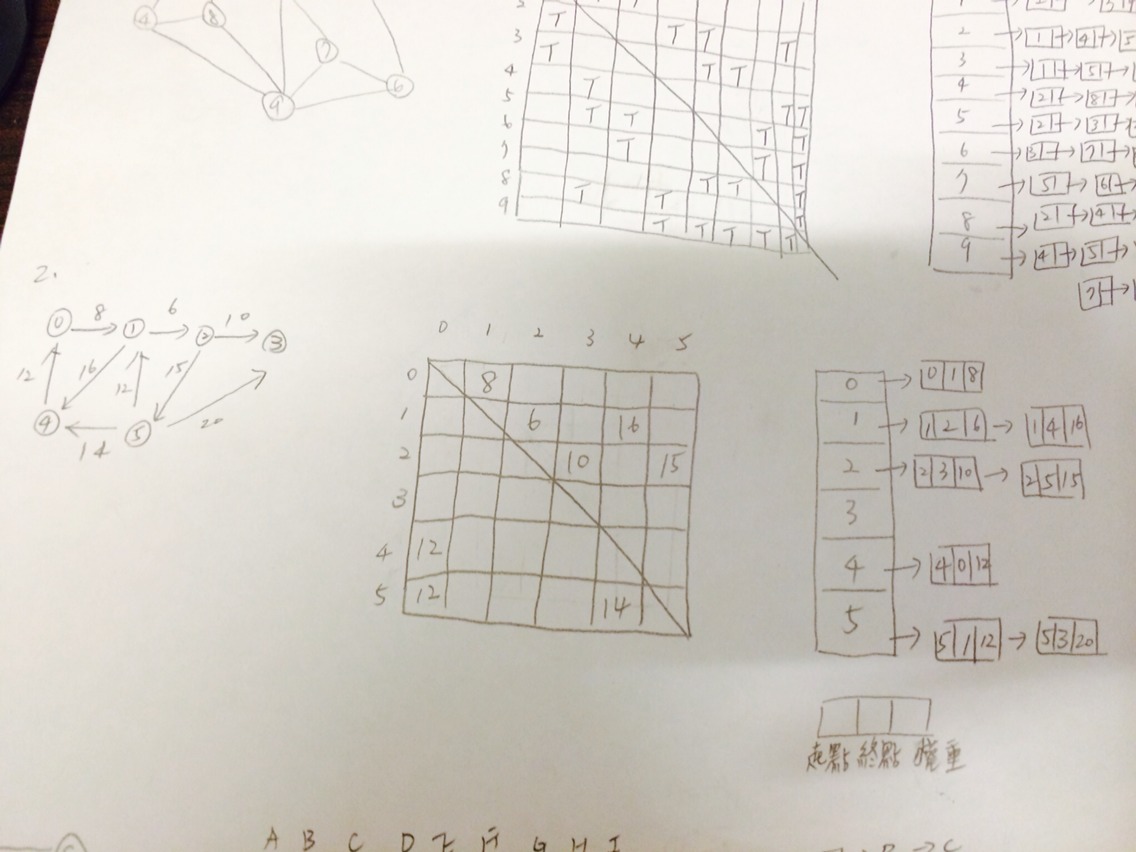This black and white image features a detailed mathematical equation involving a grid system. Within the grid, various data points are connected by arrows, indicating a series of relationships or steps in a problem-solving process. The entire composition is rendered in pencil or pen, emphasizing its hand-drawn and analytical nature. On the right side of the grid, a column labeled with numbers 0 through 5 is present, each number accompanied by an arrow pointing to a sequence of numerical values such as 0, 1, 8, 1, 2, 6, 1, 4, 6. This arrangement suggests that the image is capturing a detailed moment of complex mathematical computation or algorithmic representation.